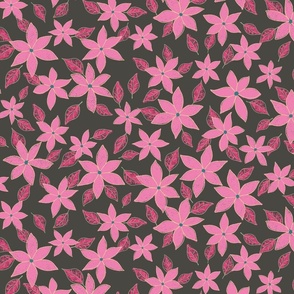This image features a striking arrangement of bright pink flowers with six long, teardrop-shaped petals, each having a green center. These flowers densely cover the dark, almost black background, creating a bold contrast. Underneath the flowers, some oval-shaped leaves are visible; they are darker in color with white veins and outlines, adding depth to the image. The overall effect is akin to a detailed, hand-drawn illustration or sophisticated wallpaper, with the vivid pink hues of the blooms and leaves standing out prominently against the backdrop.